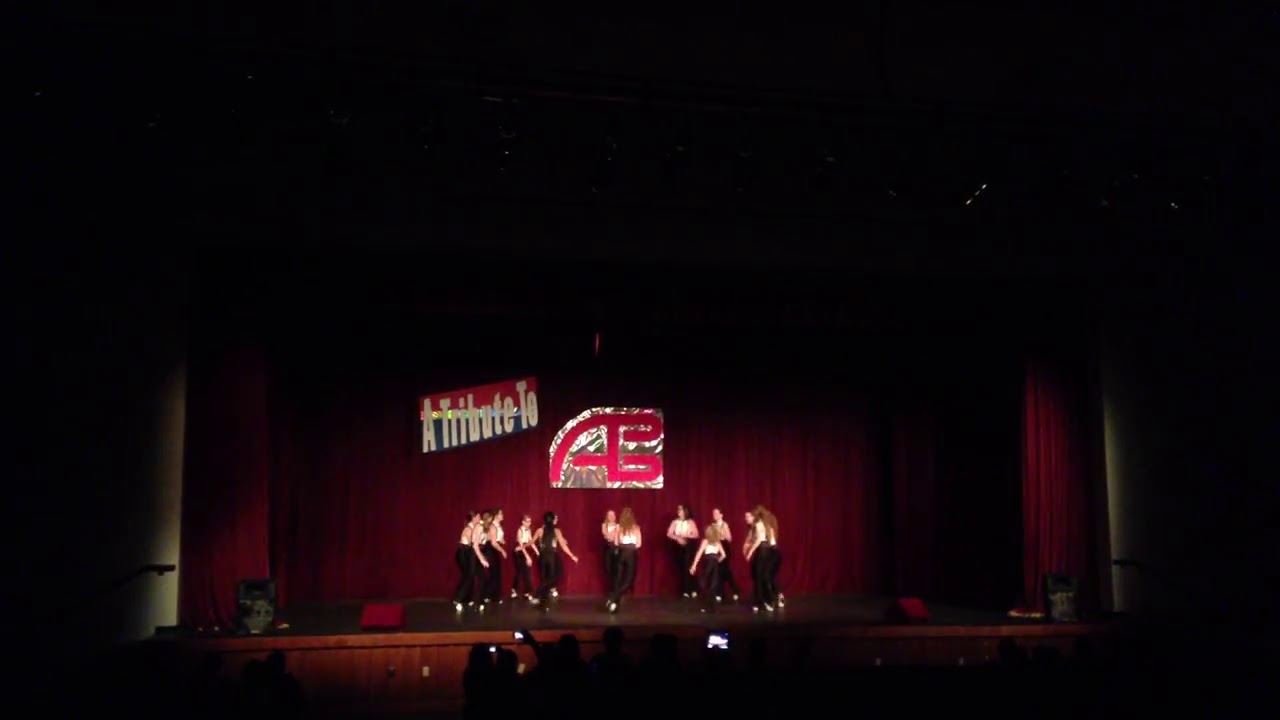In a dimly lit auditorium, the image captures a stage performance set against a backdrop of rich red curtains. The focal point is a group of young women, approximately 10 to 12 in number, uniformly dressed in tight black pants and light-colored sleeveless tops or white blouses. One performer stands out, dressed entirely in black. The stage is adorned with a sign that reads "A Tribute to A.B.," accompanied by an emblem reminiscent of the American Bandstand logo, a nod to the iconic TV show once hosted by Dick Clark. The scene is framed by the red drapery pushed to the sides, revealing the vibrant stage in contrast to the surrounding darkness. Silhouettes of the audience, some with phones raised to capture the moment, mark the bottom edge of the photo, accentuating the performers in the spotlight. Hints of stage lighting can be seen as small specks above, contributing to the overall atmosphere of an ongoing performance.